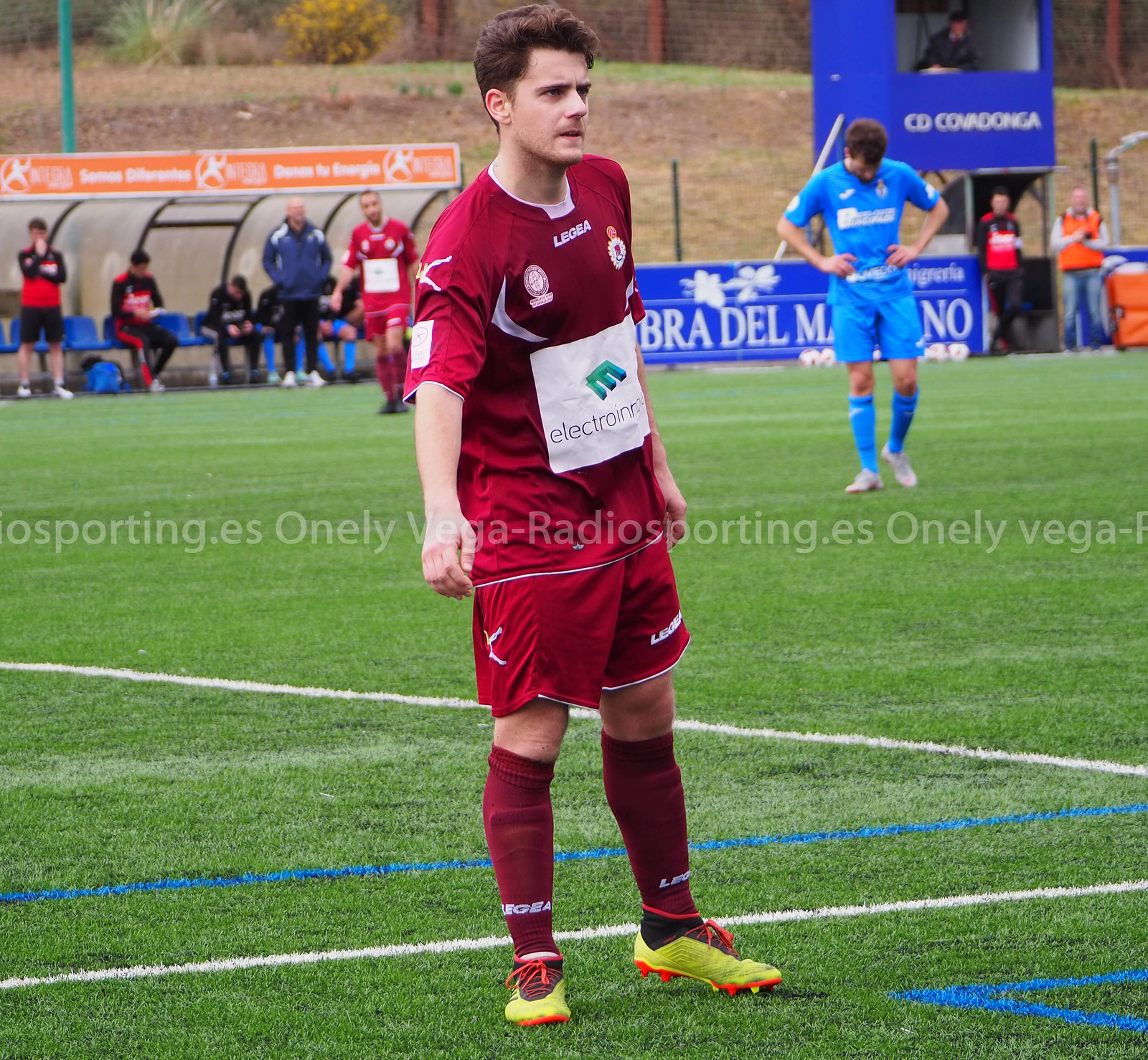The image captures an outdoor soccer game on a vibrant green field, marked with both white and blue lines. In the foreground, a fair-skinned player with mid-length brown hair is prominently featured, donning a red jersey, red shorts, and tall red socks. His striking neon yellow-green cleats with neon orange laces and studs draw attention. Positioned behind him is another player in a blue jersey, blue shorts, and blue socks, wearing white cleats. This player appears contemplative or fatigued, with his head bowed slightly. Additionally, there is a third player in the middle ground wearing a blue kit. The image features a background with signage in Italian and showcases spectators, teammates, and a coach in a blue windbreaker. A shelter with blue seats is also visible, housing several individuals either sitting or standing nearby. The scene is accented with a translucent overlay text reading "wanli vega-radiosporting.es," repeated across the picture.